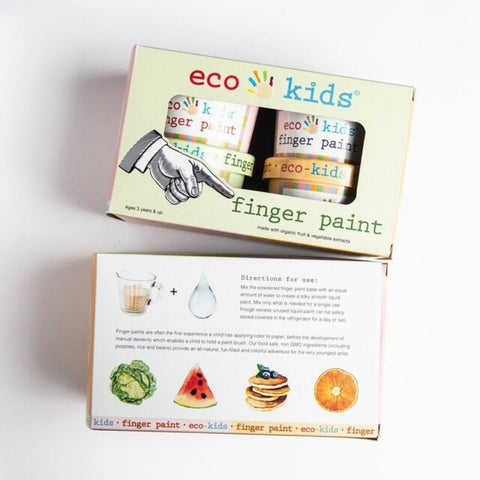The image displays two boxes of children's finger paint positioned against a white background, casting natural shadows that emphasize the photograph's authenticity. The upper box showcases its front side, featuring an ivory color with "Eco Kids" at the top, accompanied by an image of a small, white hand with each finger dipped in paint. Below this, a black and white illustration of a finger points towards the words "finger paint" in the bottom right corner. The center of the front box is open, revealing four small eco-friendly finger paint pots labeled "Eco Kids Finger Paint."

The lower box reveals the back side, which is predominantly white. It includes a visual of a measuring cup and a large drop of water, adjacent to "Directions for Use" written in black text followed by explanatory details. The center section contains additional black writing. At the bottom, illustrations of a head of lettuce, a watermelon slice, a stack of pancakes with blueberries, and an orange slice are depicted. An ivory banner at the base of the box reads "Kids Finger Paint, Eco Kids Finger Paint, Echo Kids Finger." Overall, the cohesive details across both boxes emphasize the product's child-friendly and eco-conscious design.